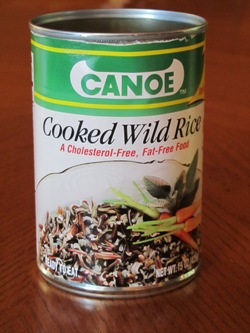A close-up image of a can is displayed, tilted 90 degrees to the right on a smooth, polished wooden table. The can, branded "Canoe" (C-A-N-O-E), features the brand name in green letters on a white banner, itself set against a green background adorned with two thin yellow stripes. In the bottom right corner of the white banner, there is a "TM" designation. 

Below this design, the can transitions to a white section featuring black text that reads "Cooked Wild Rice." Further down, red text proclaims the contents to be "A cholesterol free, fat free food." At the bottom of the can, an image of the food showcases brownish wild rice accompanied by full carrots with green stalks, all presented on a plate. To properly view the image, one would need to tilt their head 90 degrees to the right.